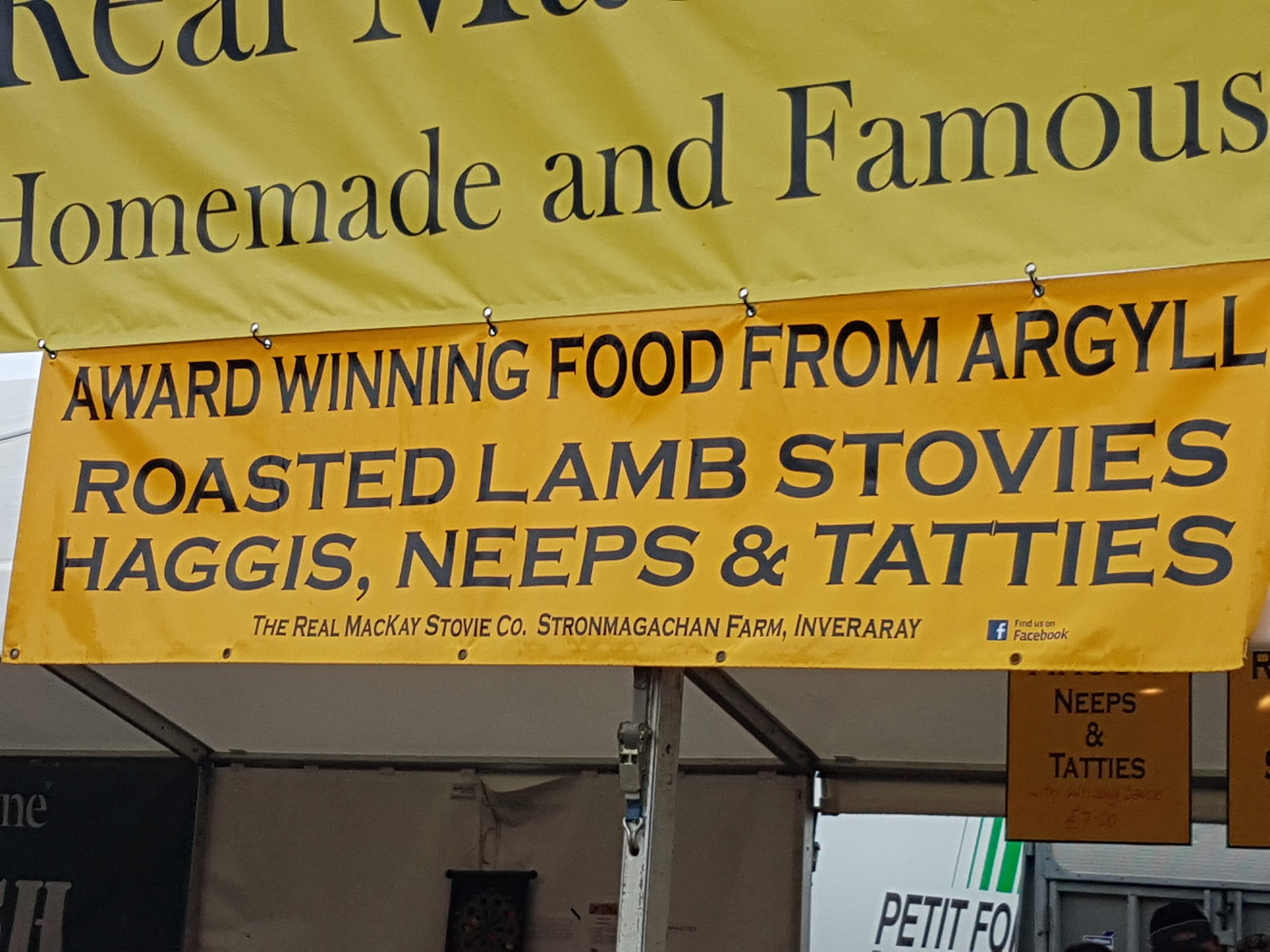This is an outdoor photograph of a food concession stand, featuring two yellow-hued banners affixed to an overhang. The top banner, in a light yellow color, partially reads "Homemade and Famous" with some of the text obscured. The lower, dark yellow banner displays detailed information about the offerings: "Award-winning food from Argyll - roasted lamb, stovies, haggis, neeps, and tatties." The banner attributes these delicacies to "The Real MacKay Stovie Co." from "Strong Market Sean Farm, Inveraray." The banners are held up by metal supports and appear to advertize a Scottish food vendor, emphasizing their recognition and traditional dishes.